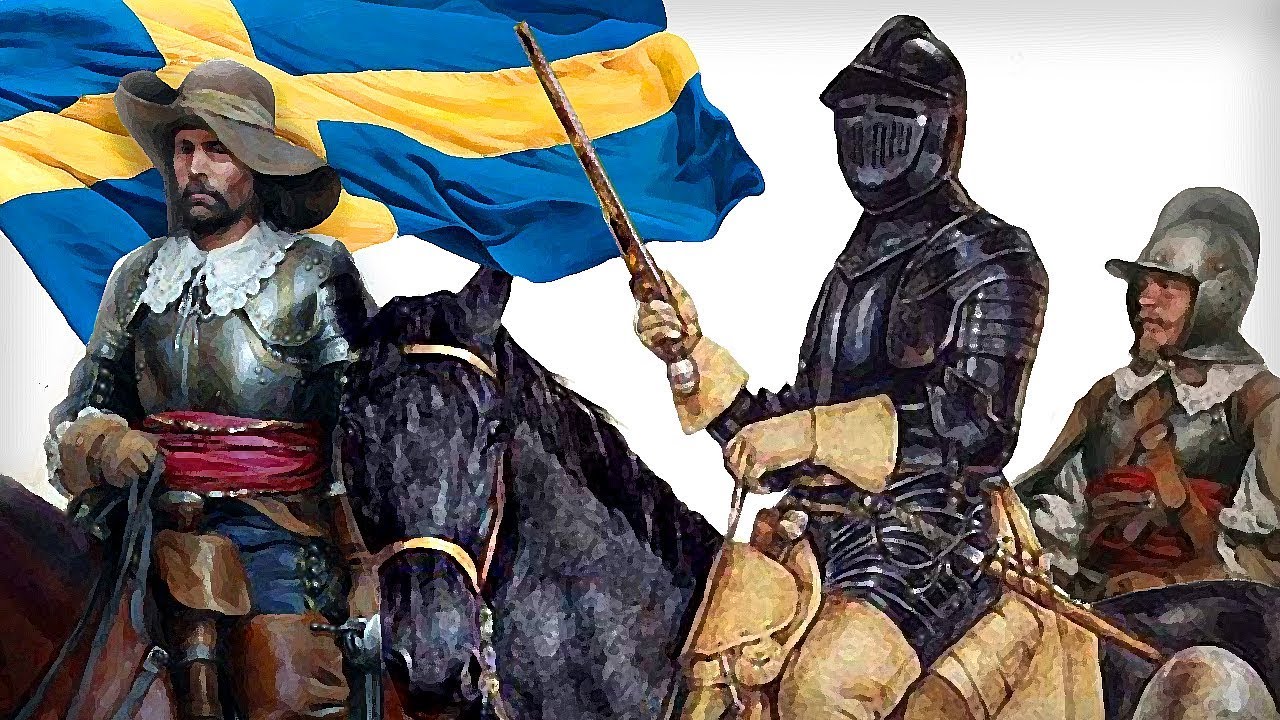In this detailed oil painting or drawing, depicted with a white background, the central focus is three men on horseback in front of the flag of Sweden, seen in the upper left-hand corner. The man on the far left rides a brown horse while wearing chest armor paired with an unusual lace top and a brown floppy hat. His distinct appearance is completed by the fact he holds the Swedish flag. The central figure is depicted as a full-fledged knight in dark gray, almost black armor that covers his entire body, including his head and face. He manages the reins with his left hand and holds a weapon in his right. The man on the right, although his horse is not fully visible, is situated at the same level, indicating he is also mounted. He sports a protective helmet, different in style as it leaves his face visible, and has a silver-toned breastplate. The overall scene merges elements of both medieval and possibly even cowboy aesthetics.